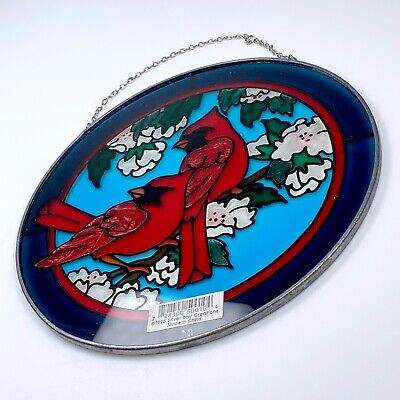The image displays a round stained glass wall hanging, slightly tilted from the top right to the bottom left corner, suspended by a silver chain. The hanging features two vividly red cardinal birds with dark, black-tinted faces perched on a brown branch. Surrounding the birds are green leaves and delicate white flowers, all set against a serene blue sky background. The outer edges are dark grey, bordered by a dark blue band, while a red border encircles the painting at the center. Notably, there is an ISBN barcode visible on the back, indicating it as a purchasable item.